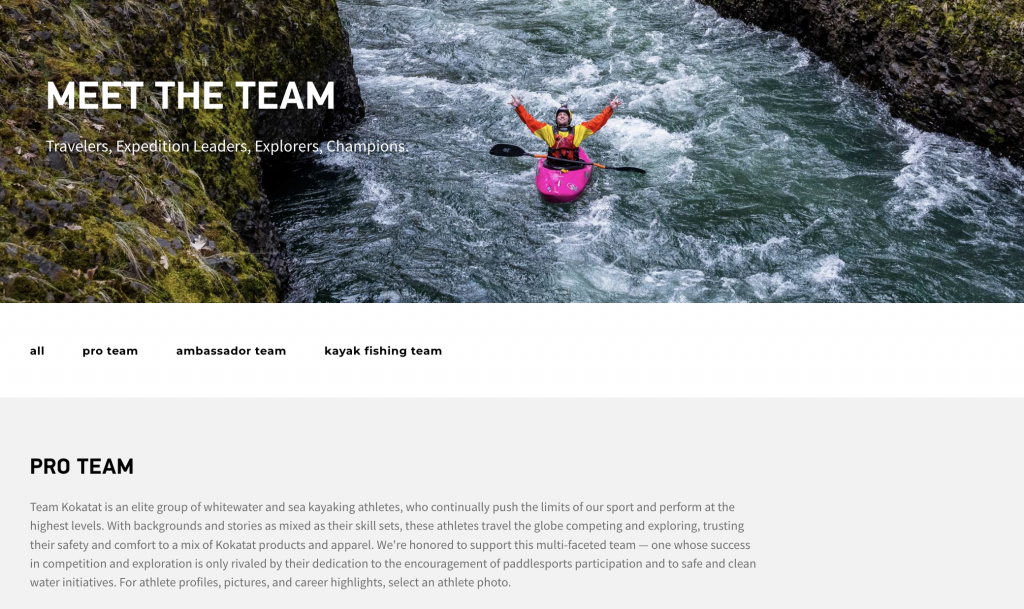At the top of the image, a person in a pink kayak navigates through challenging river rapids, with cliffs rising majestically on either side. The image is adorned with text that reads: "Meet the Team - Travelers, Expedition Leaders, Explorers, Champions. All-Pro Team, Ambassador Team, Kayaking and Fishing."

Below the image, set against a gray box with black font, a detailed description highlights the elite group of whitewater and sea kayaking athletes. The text elaborates on their relentless pursuit of pushing the limits of their sport and performing at the highest levels. It mentions that these athletes come from diverse backgrounds and possess various skill sets, united by their commitment to competing and exploring around the globe. The athletes rely on a blend of products and apparel for their safety and comfort during their adventures.

The caption continues to emphasize the honor and support given to this versatile team, noting that their success in both competition and exploration is matched by their dedication to promoting paddle sports, participating in initiatives for clean and safe water, and showcasing athlete profiles, pictures, and career highlights. A call to action invites viewers to "Select an Athlete Photo" for more information.